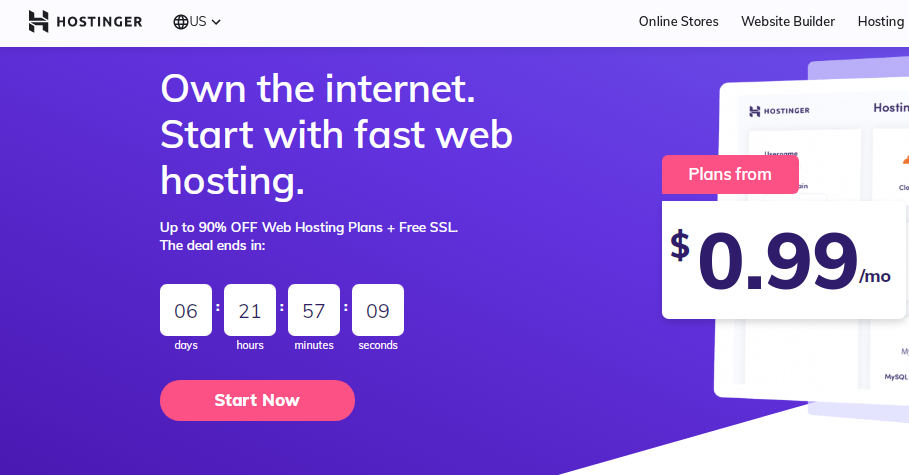The image depicts an advertisement for Hostinger's monthly plan, prominently displayed on a website. In the upper left-hand corner, the Hostinger logo, a black "H" symbol, is positioned next to the brand name "Hostinger" spelled out in white text. Adjacent to this, there is a globe icon labeled "US" with an accompanying drop-down menu.

To the right, a gray navigation bar features links titled "Online Stores," "Website Builder," and "Hosting." Below this navigation bar, the background transitions into a dark purple section, primarily filling the rectangular space. A white gradient accent is present in the bottom right-hand corner of this purple area.

Centralized in this dark purple portion, bold white text reads: "Own the Internet, Start with Fast Web Hosting, up to 90% off web hosting plans plus free SSL." Below this, a countdown timer indicates the deal's expiration in 6 days, 21 hours, 57 minutes, and 9 seconds. Beneath the timer, a striking pink button with white text invites users to "Start Now."

To the right of this central message, additional promotional text highlights that hosting plans start "From $0.99 a month."